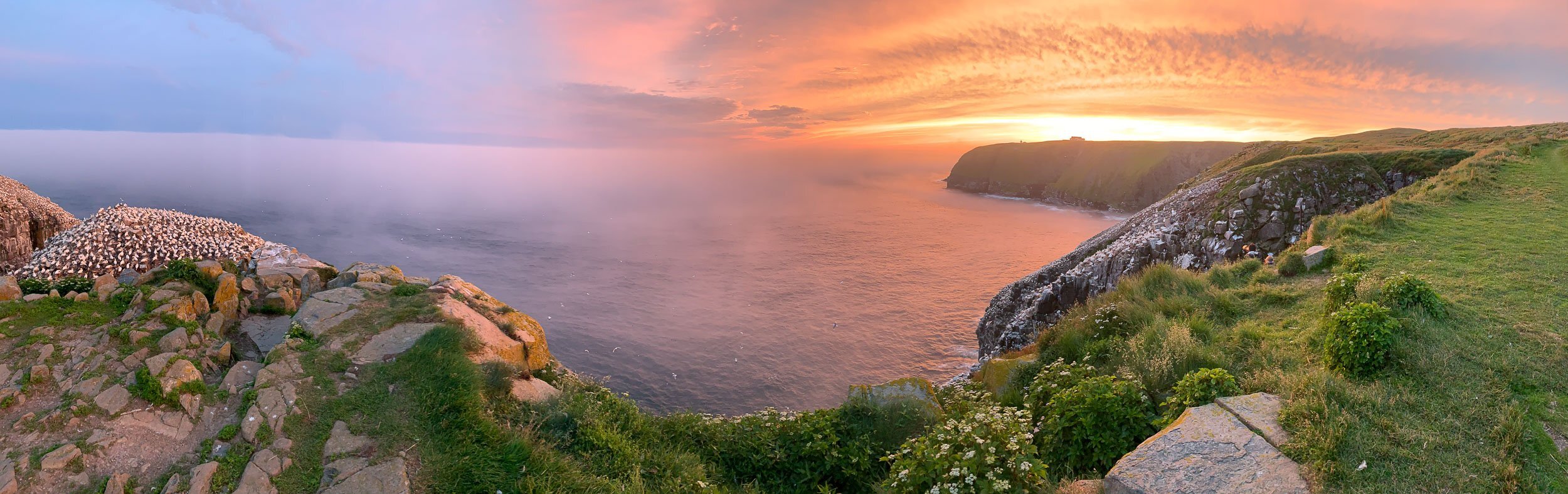This captivating image showcases a serene and scenic landscape that could be representative of Ireland. It captures the moment of a sunrise or sunset over a rocky cliff shoreline. The cliff is lush and green, with vibrant grass, green plants, and shrubs adorned with white flowers. The tan-colored stones, some dusted with white powder, add texture to the scene. Below, a vast expanse of either an ocean or a large body of water stretches out, slightly misty or foggy at the horizon. The sun, either rising or setting, paints the sky in stunning hues of yellow and orange, contrasting with the blue of the clearer sky. Bands of clouds, tinged golden, float above, adding to the tranquil and picturesque panorama. The steep drop from the cliff's edge to the water emphasizes the dramatic and breathtaking nature of this beautiful, tranquil setting.